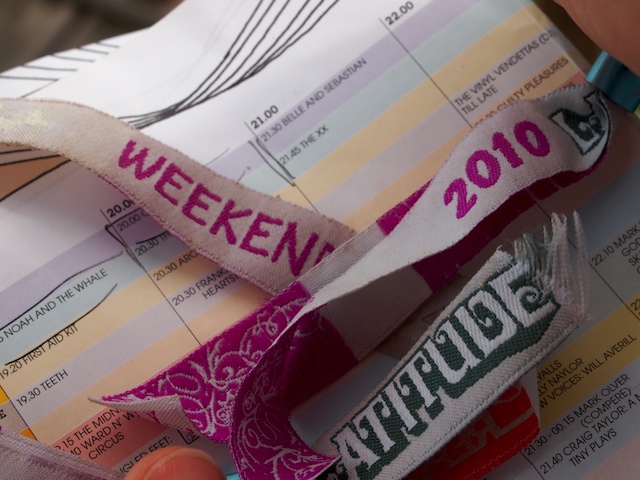The image depicts a chaotic tabletop scene. A variety of colorful pieces of fabric and paper dominate the view. On the left, a piece of white fabric with uppercase purple text spelling out "WEEKEND" hangs down toward the center. An intricate pink fabric piece extends diagonally from the bottom left, featuring white lines that transition between pink and white sections. Above this fabric, there's a lanyard with a white background and "2010" printed in blue and pink, followed by another fabric piece labeled "ATTITUDE" in white text with a green shadow, surrounded by strings waving upward.

Below these fabrics lies a cluttered array of papers highlighted with various colors and black writing. The papers display sections with printed numbers 20 to 22 and charts. In the topmost purple section, "2130 Bella and Sebastian" is noted. A light green row beneath it lists "21 to 45 The XX" and "Noah and the Whale" along the left side. A yellow section below includes "1920 First Aid" and "2030 ARC." At the bottom, a light purple row reads "1930 Coal and Teeth," and next to it, "2030" is partially obscured by fabric. In the upper right corner, the words "The Vinyl Venetians" appear, partially cut off, followed by "till late."

The scene overall suggests a mix of personal items and paperwork, possibly related to an event or festival, with notable bands and times circled such as "Noah and the Whale," "First Aid Kit 1920," and "Teeth 1930." The vibrant wristbands and lanyards hint at a lively, yet cluttered, snapshot of someone's organizational system for an eventful day.